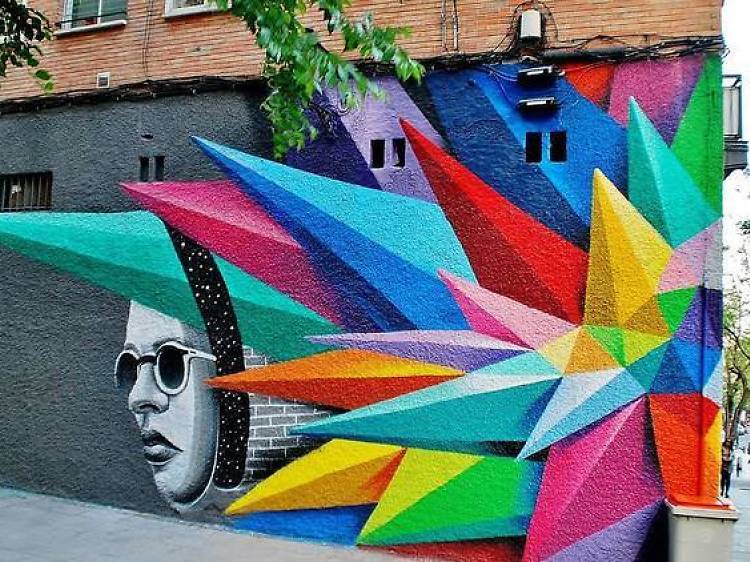This photo captures a vibrant and intricate mural painted on a textured gray concrete wall outside a business on a sidewalk. The mural is a stunning array of 3D-looking, colorful triangular prisms and pyramids, resembling spiky gemstones or origami, jutting out in various vivid colors including red, orange, yellow, green, blue, purple, and pink. Each prism is uniquely shaded, adding to the illusion of depth. 

On the left side of the mural, emerging from these angular shapes, is the serene face of a woman wearing white sunglasses, depicted in gray. Her face is positioned towards the bottom left, with a black line resembling the night sky leading to it. The rest of the wall is freshly painted gray, providing a neutral backdrop for the colorful artwork. Above this gray-painted portion, the top of the building is made of red brick, with a few small tree branches hanging down. In the bottom right corner, a garbage can is visible, and a few people can be seen walking in the background on the right side. 

This mural transforms the ordinary urban landscape into a striking visual experience, making passersby pause and marvel at its complexity and beauty.